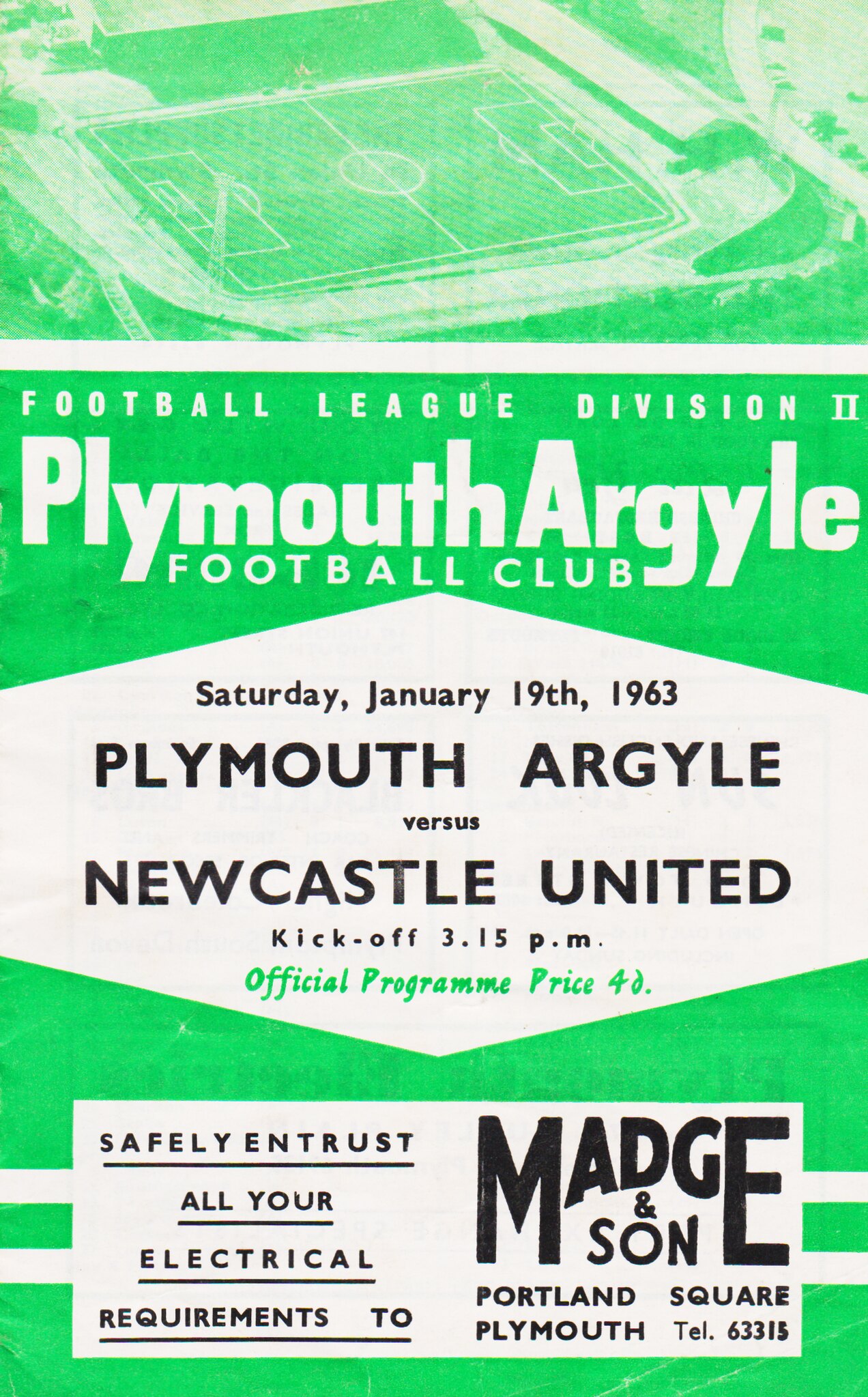The cover of the magazine or sports program is predominantly green with sections of white and black text. At the top of the cover, it features an artist’s rendition of an aerial view of an empty soccer stadium, with the stadium structure depicted in white against the light green background. Below this illustration, there is a green banner with white text that reads "Football League Division II Plymouth Argyle Football Club." 

A white diamond is centrally situated on the cover, containing black text that states the match details: "Saturday, January 19, 1963, Plymouth Argyle vs. Newcastle United. Kickoff, 3.15pm." Further down, green text indicates the publication's official nature: "Official Program Prize for D." The lower section of the cover includes more black text and features an advertisement advising to "Save and trust all your electrical requirements to brand name." 

Overall, the composition and colors create a vibrant and clear presentation of the soccer event details and related information.